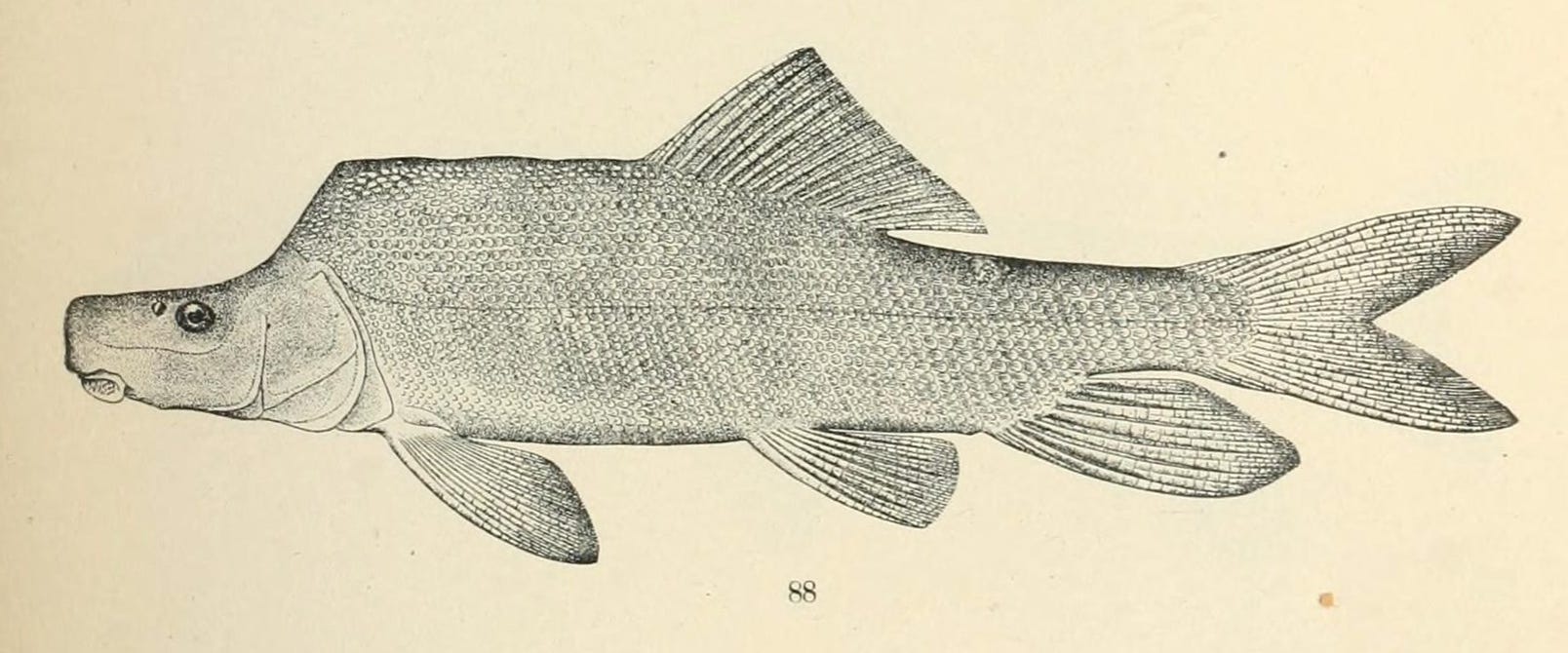This is a detailed grayscale illustration, reminiscent of a pencil drawing, featuring an unusual fish on a cream-colored, aged, and yellowed page marked with the number 88 at the bottom center, indicating it's from a book. The fish is strange-looking and likely not common; it could be fictional, prehistoric, or extinct. Oriented horizontally with its head pointing to the left, this fish has a bizarre, snout-like head with an eye positioned on the snout and a sucker's mouth filled with teeth-like features. Its body, much larger than its head, is intricately detailed with meticulously drawn scales. The fish possesses three fins extending from its underside, one dorsal fin at the top, and a forked tail. There is also a blot or possibly some gold and yellow mark at the bottom right of the image, adding to the aged appearance of the page.